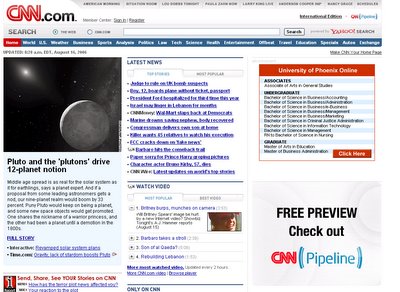The webpage features the CNN logo prominently at the top left, with "CNN" in red lettering and ".com" in black lettering. The header includes several categories against a gray background, though they are too zoomed out to be legible. Below the header, a centered search bar is flanked by "Yahoo" in red text on the right. 

The main body of the page comprises a blue strip with 10 to 12 categories listed in white text. The leftmost section sports a red background with the word "Home" displayed. Beneath this is an article titled "Pluto and the Plutons Drive 12 Planet Notion," accompanied by an image of a planet in space. A paragraph of text and multiple links follow the image.

In the central section, there's a list of links in blue text under the heading "Latest News". On the right, another red background features the text "University of Phoenix Online," followed by several sentences in black. At the bottom-right corner, there's a free preview section titled "Check Out CNN (Pipeline)" in blue text set against a light gray and white fused background.